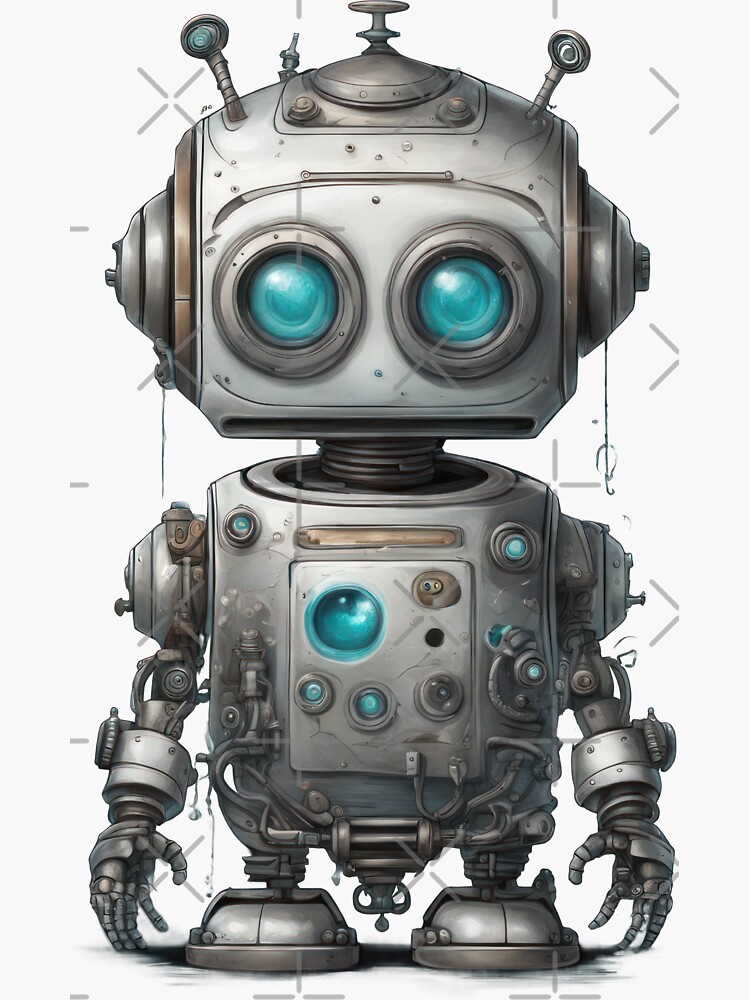This detailed illustration portrays a charming, retro-futuristic styled robot set against a clean, stripped white background, giving it a standing-out effect. The robot features an oversized head adorned with two small antennae and swirly, marble-looking turquoise eyes that convey an inviting, friendly demeanor. The head is further detailed with bolts and nuts resembling ears and a cute smile. Its body is a grayish metallic hue, richly textured with pipes, wires, and various metallic details. Its torso is prominent, featuring five circular elements on the belly, one notably large and turquoise, with the others being gray with turquoise accents. The humanoid arms are crafted with a mix of metal straps, cork-like joints, and screws, extending all the way to its short metallic feet, making it appear as though it would shuffle along when moving. The overall design, potentially created digitally or painted, evokes a nostalgic, yet endearing robotic character. Additionally, the image is watermarked with cross-hatched X's, heightening its crafted aesthetic.